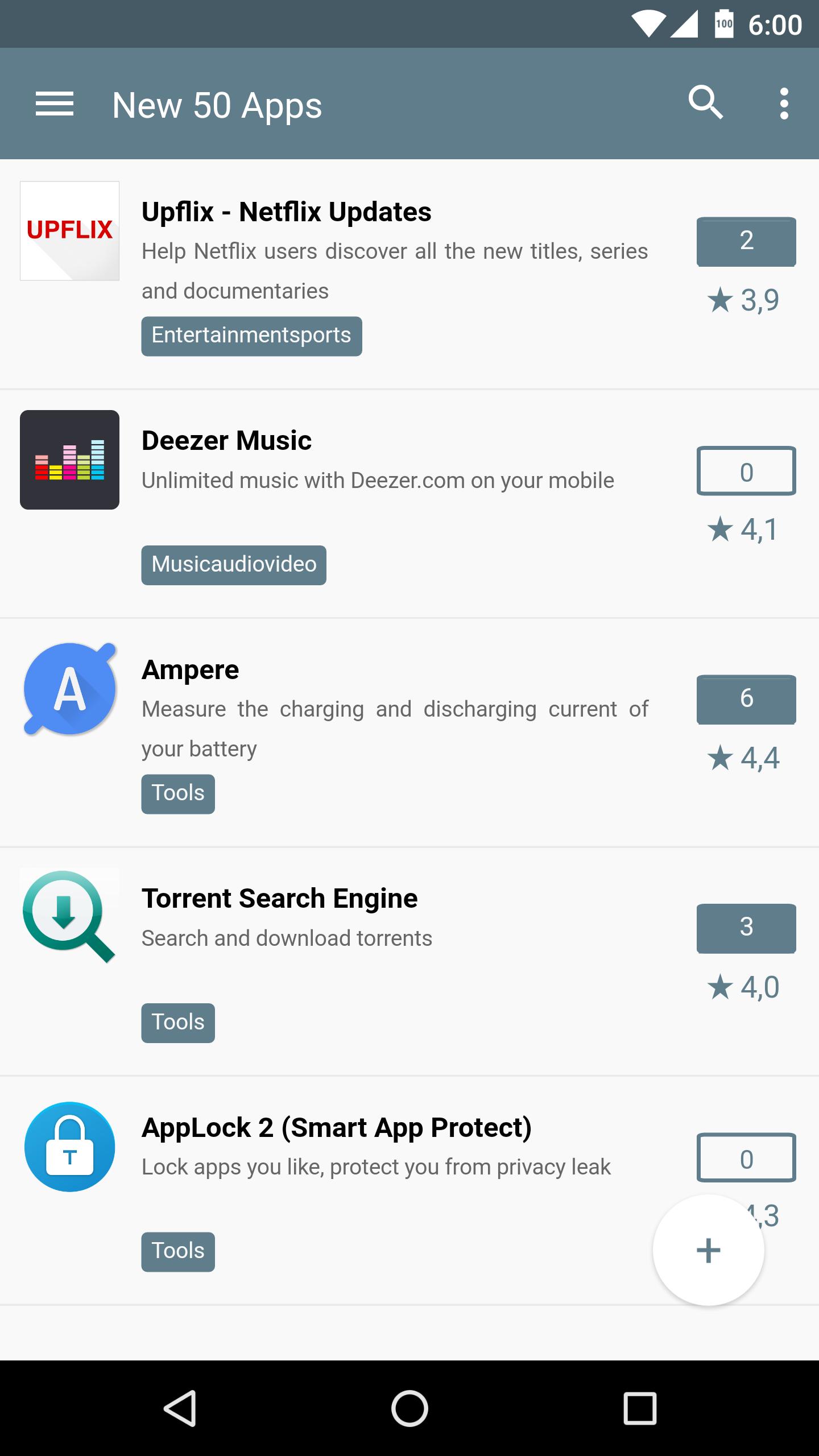The image is a detailed screenshot of a mobile application taken at 6 o'clock. The phone displays a full 100% battery life, complete carrier signal bars, and an active Wi-Fi connection. Within the app, we can see a notification stating "New 50 apps" alongside a magnifying glass icon for search functionality.

The main screen showcases three featured apps with detailed descriptions:

1. **UpFlix**: Presented with a white background and red text in a square icon, UpFlix is an app designed to help Netflix users discover new titles, series, and documentaries. A blue box with the number 2 signifies its ranking or another category indicator. The app has a rating of 3.9 stars, with blue-colored stars. It's categorized under "Entertainment" and "Sports."

2. **Deezer Music**: This app is symbolized by a black square containing a multi-colored musical graph (red, yellow, and blue). It offers unlimited music streaming via Deezer.com on mobile devices. Deezer Music boasts a rating of 4.1 stars, also in blue. Categories for this app include "Music," "Audio," and "Video."

3. **Ampere**: Featuring a circular icon with the letter "A," Ampere measures the charging and discharging current of your battery. The app is highly rated with 4.4 stars, with the rating stars colored blue.

Each app description is accompanied by respective star ratings and their color-coded categorizations, making it easy for users to identify and decide on downloads.